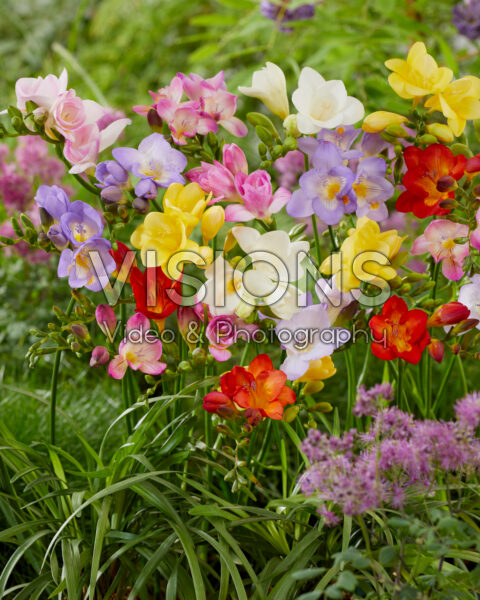This image features a vibrant, close-up view of various types of flowers in a natural setting, possibly a field or garden. Dominating the center in a horizontal band, the flowers display a stunning palette of colors, including shades of white, pink, light purple, orange-red, red with touches of yellow, solid yellows, and bright pinks. Among the different varieties, freesia and roses can be identified. The foreground and background are lush with greenery, including tall grass that blends with the flower stems. The grass also has purplish hues, adding to the rich tapestry of colors. Superimposed over this lively scene is a transparent watermark reading “Visions Video and Photography,” with the word "Visions" appearing larger and higher than "Video and Photography" beneath it. No people or additional text are present in the image besides the watermark.